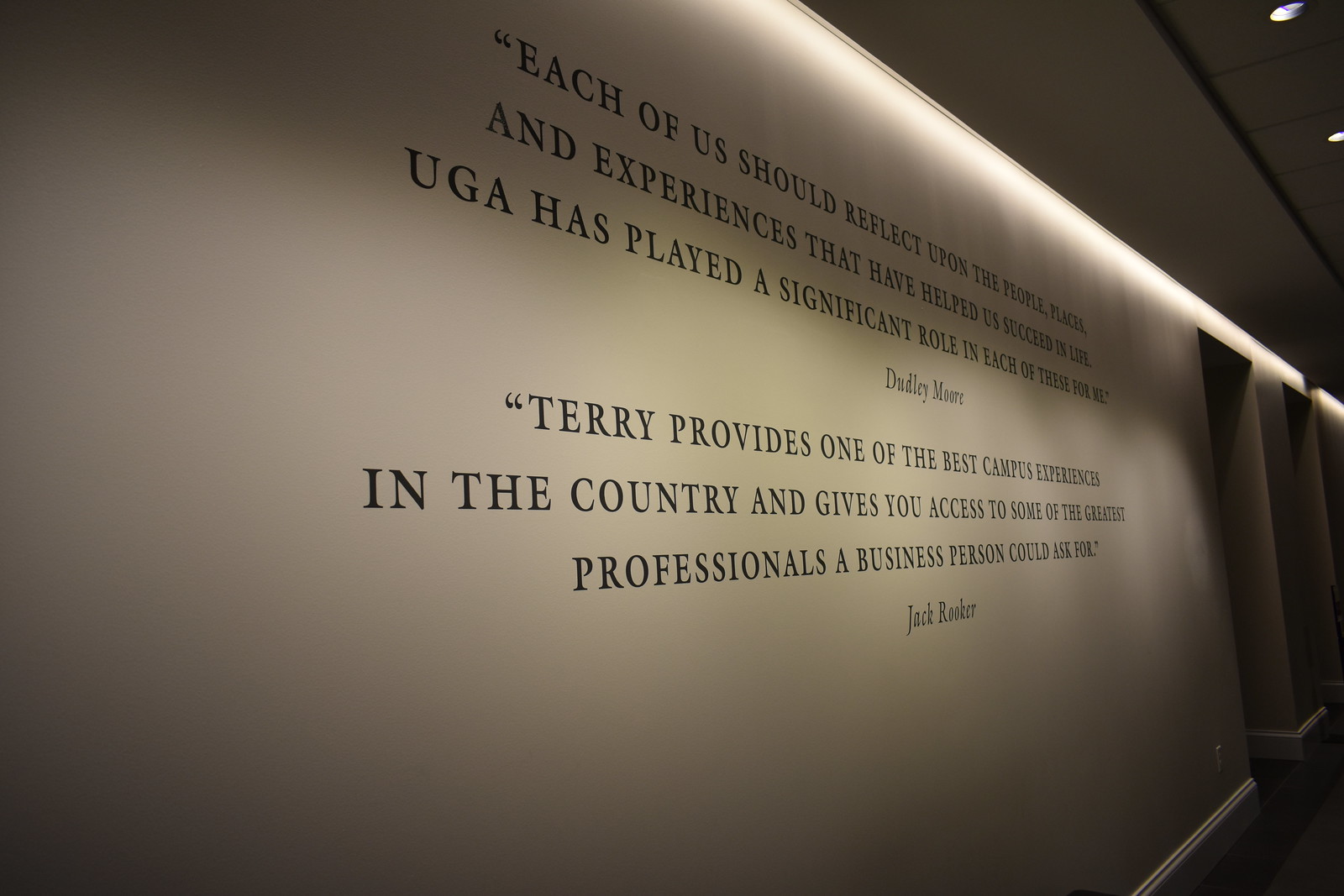The image captures a dimly lit hallway in a museum, presenting a detailed look at a prominent billboard. The hall features white walls, with doorways leading to other sections, under a subtle lighting strip that partially illuminates the space. The photograph is taken from the left side, giving a slightly oblique view of the text on the billboard. The text consists of two quotes, the first of which reads, "Each of us should reflect upon the people, places, and experiences that have helped us succeed in life. UGA has played a significant role in each of these for me," attributed to Dudley Moore. The second quote states, "Terry provides one of the best campus experiences in the country and gives you access to some of the greatest professionals a business person could ask for," credited to Jack Rooker. The interplay of light and shadow on the billboard accentuates parts of the quotes while leaving other parts in darkness, adding a dramatic effect to the portrayal of these impactful messages.